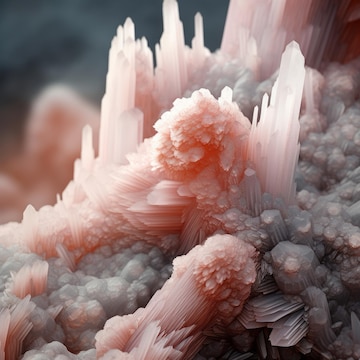The image presents an otherworldly, abstract crystal formation dominated by various shades of pink and gray. The central structure features numerous crystal shafts rising in multiple directions, some clustering to form sharp spikes, and others appearing lumpier and less defined. The composition showcases a gradient from a rose pink to pale pink, with interspersed gray tones, creating a striking contrast. The base of the formation is predominantly gray, transitioning to pink as the crystals ascend. The background is blurred, emphasizing the intricate and somewhat surreal details of the crystal structures, which evoke the appearance of an alien landscape or an underwater spectacle captured under a microscope.